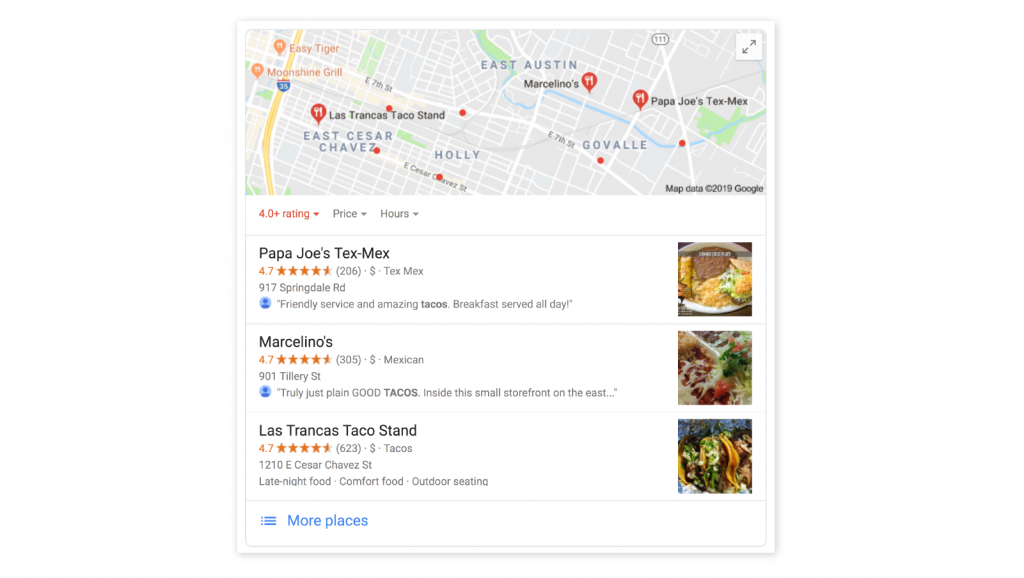The image depicts a Google Maps interface focused on East Austin, featuring key roads like Cesar Chavez, Holly, and Govalle Avenue. The user appears to be searching for highly-rated dining options, specifically those with at least a 4.0-star rating. 

The first highlighted restaurant is Papa Joe's Tex-Mex, located at 917 Springdale Road. It boasts friendly service, amazing tacos, and serves breakfast all day. 

The next recommendation is Marcelino's, with a 4.5-star rating, situated at 901 Tillery Street. This quaint eatery is praised for its straightforward but delicious tacos served within a cozy storefront.

The final venue listed is Las Trancas Taco Stand, which enjoys a 4.7-star rating and can be found at 1210 East Cesar Chavez Street. Known for its late-night and comfort food offerings, this spot features an inviting outdoor setting.

Each restaurant is accompanied by tantalizing images of their food plates, making the options even more appealing.